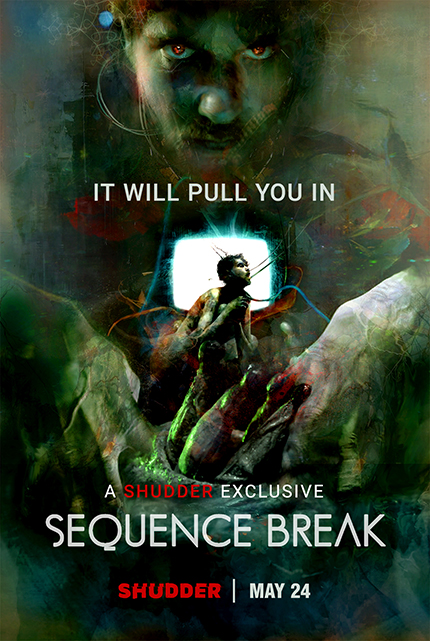This is an advertising poster for a Shudder exclusive, a television show or possible gaming announcement titled "Sequence Break," premiering on May 24th. The poster is predominantly green and black, creating a dark and eerie atmosphere. At the top center, it features a menacing face with red eyes, exuding a sinister aura. Below this face, bloody and gory hands stretch out from both sides towards the center of the image. Positioned between these hands is a figure shrouded in wires, appearing to be in agony, standing in front of a large, glowing, old-style television screen. The tagline at the top reads, "It Will Pull You In," and the overall design of the poster is both unsettling and captivating, combining elements of horror and suspense.